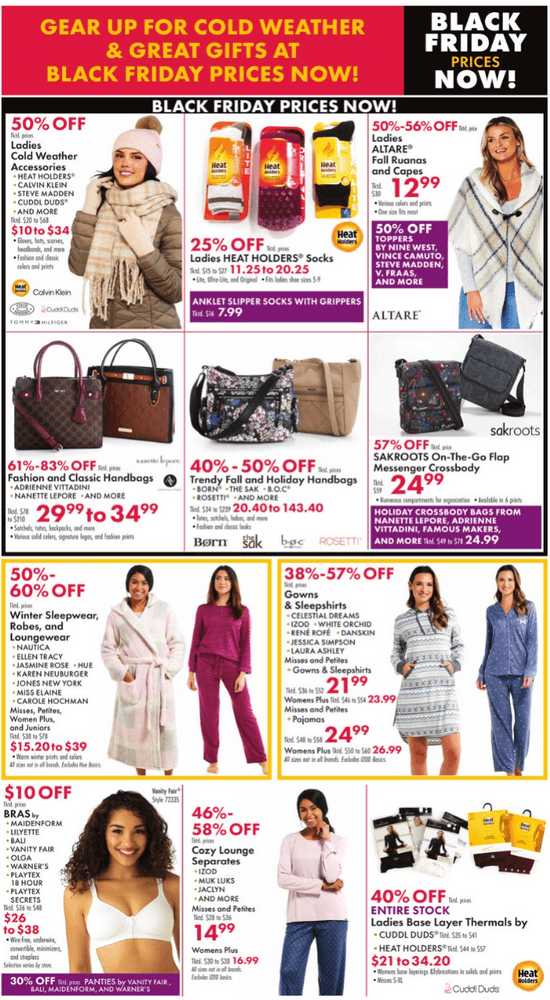In portrait format and vibrant color, this advertisement, likely photographed from a free coupon magazine, is a visually bustling array of Black Friday deals. The top right corner boldly announces, "Black Friday prices now," enticing viewers with the promise to "gear up for cold winter weather and great gifts at Black Friday prices now." The ad is densely packed with images and discounts, showcasing a variety of winter essentials and gift ideas.

Prominently featured is a young, stylish woman in her twenties, adorned in cozy winter attire—hat, gloves, and a substantial jacket, advertising "50% off ladies cold weather accessories." Next to her, a deal showcases "25% off ladies heat holder socks," complete with an image of the thick, warm socks. The ad continues with "50% to 56% off ladies' all-terrain fall Ruanas and capes," alongside appealing images of these fashion items.

Additional discounts extend to a wide array of products, including fashion and classic handbags, winter sleepwear, robes and loungewear, gowns and sleep shirts, and bras, all pictured to entice potential buyers. This meticulously organized layout maximizes the available space, cramming in as many appealing offers as possible, making it a quintessential example of a holiday-themed, value-packed advertisement.